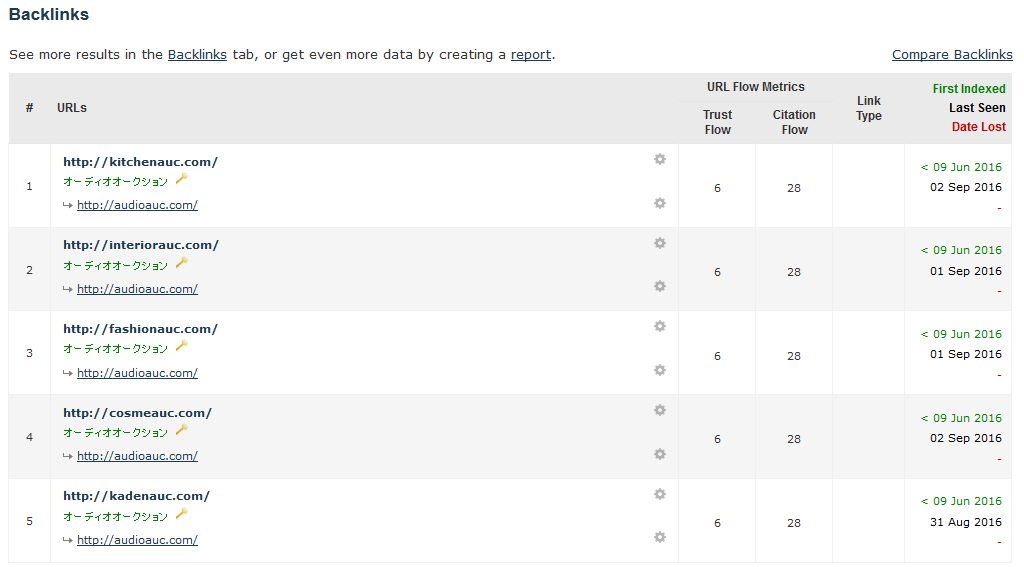The image displays a detailed interface focusing on website backlinks, with various interactive elements and metrics. In the top left corner, the word "Backlinks" is prominently displayed. Beneath this, there are clickable options: "See more results in the Backlinks" and "Get even more data by creating a report," both underlined for emphasis. The main section of the image has a gray shaded area containing a table with multiple columns labeled "Number," "Icon," "URLs," and "URL Flow Metrics." 

To the right, the "URL Flow Metrics" section includes categories such as "Trust Flow," "Citation Flow," "Link Type," "First Indexed," "Last Seen," and "Date Lost." The table lists five different backlinks, each showing uniform citation flow metrics, curiously all rated at 28. The dates associated with these backlinks range from June 9, 2016, to as late as September 1, 2016.

Below each hyperlinked web address, there is a line of Japanese text, adding linguistic variety to the listings. The entire interface is set against a clean, white background with strategically placed gray shading for visual separation and clarity.